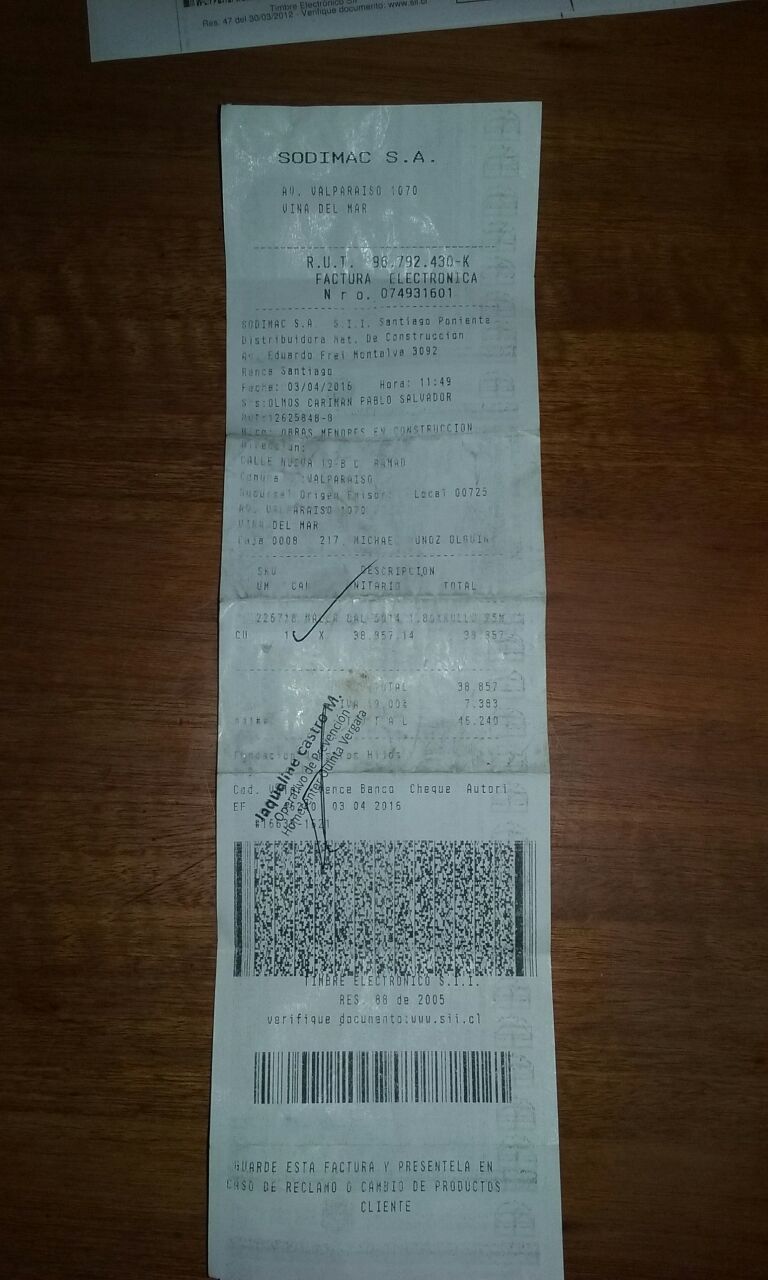The image is a color photograph of a grocery store receipt, identified as from "Sodimac S.A." The receipt, printed in black text on white paper, is laid out on a very dark hardwood table. The wood grain of the table is visibly detailed, with streaks of lighter tan colors intersecting the darker browns. The receipt features "Sodimac S.A." prominently at the top, though the rest of the text is largely illegible due to poor reflection and lighting. It appears to contain a lot of additional information, including an address: "Ava Vala Parisio 1070, Vina Del Mar." There's also a large black checkmark drawn in pen and an angled stamp reading "Jacqueline Castro M. Operativa Devo de Provincial Home Center Quinta Verga Verga." Towards the bottom of the receipt, there are two different types of barcodes: a traditional linear barcode and a QR code.